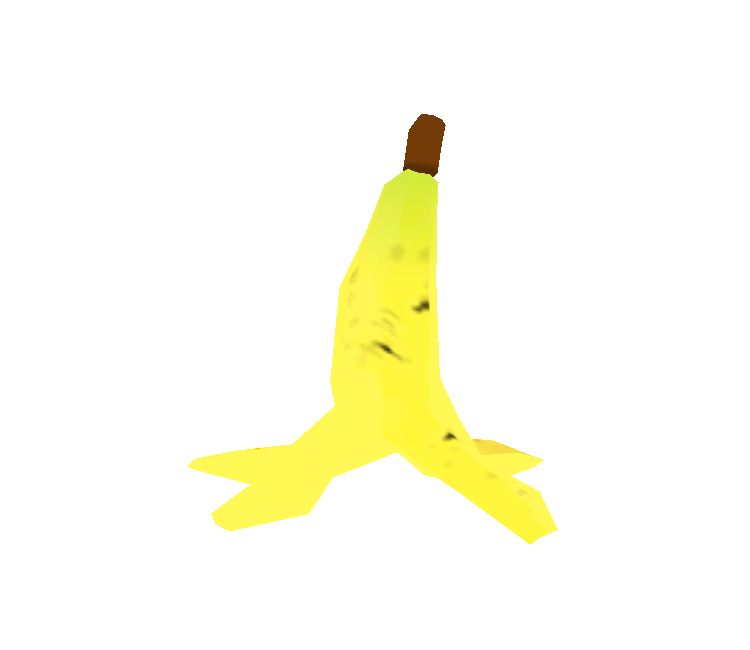The image features a low-poly, pixelated 3D rendering of a banana peel, floating in a stark white void. The digital banana peel is positioned upright in the center of the frame. Its texture is rudimentary, reminiscent of early video game graphics, such as those seen in PlayStation 1 games, with noticeable aliasing and no anti-aliasing applied. The opened banana peel has four sections splayed out, some pointing more to the left and others to the right. Its coloration transitions from a light green at the top to a rich yellow as it descends, adorned with various black spots. At the very top of the peel is a brown, cylindrical stem. The entire setup is devoid of any additional text or graphical elements, emphasizing the simplicity and digital artistry of the solitary banana peel against the uniform white background.